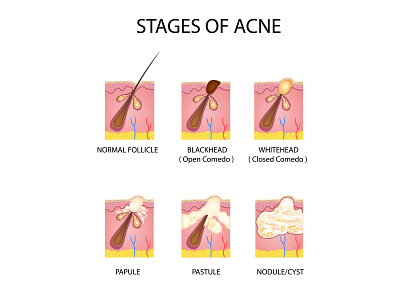This image is a detailed chart titled "Stages of Acne," presented in a six-picture grid format. The illustrations in the grid are labeled and show the progression of acne with corresponding visual representations and titles underneath each stage:

1. **Normal Follicle**: Displays a normal hair follicle with a hair strand visibly protruding from the skin.
2. **Blackhead (Open Comedo)**: Shows a blackhead at the skin's surface, representing a clogged pore where the hair should be.
3. **Whitehead (Closed Comedo)**: Depicts a closed comedo with a white or yellowish appearance where the pore is blocked.
4. **Papule**: Illustrates an inflamed lesion without pus, appearing larger and slightly raised compared to previous stages.
5. **Pustule**: Shows a more pronounced, pus-filled lesion, larger in size and a more severe form of acne.
6. **Nodule/Cyst**: Represents the most severe stage with a large, deep, and painful lesion that is entirely white, indicating significant inflammation without visible hair.

Each illustration in the grid is detailed with a cross-section view, showing a pink layer for the skin and a yellow layer at the bottom indicating deeper skin structure, along with a teardrop-shaped pore for clarity.